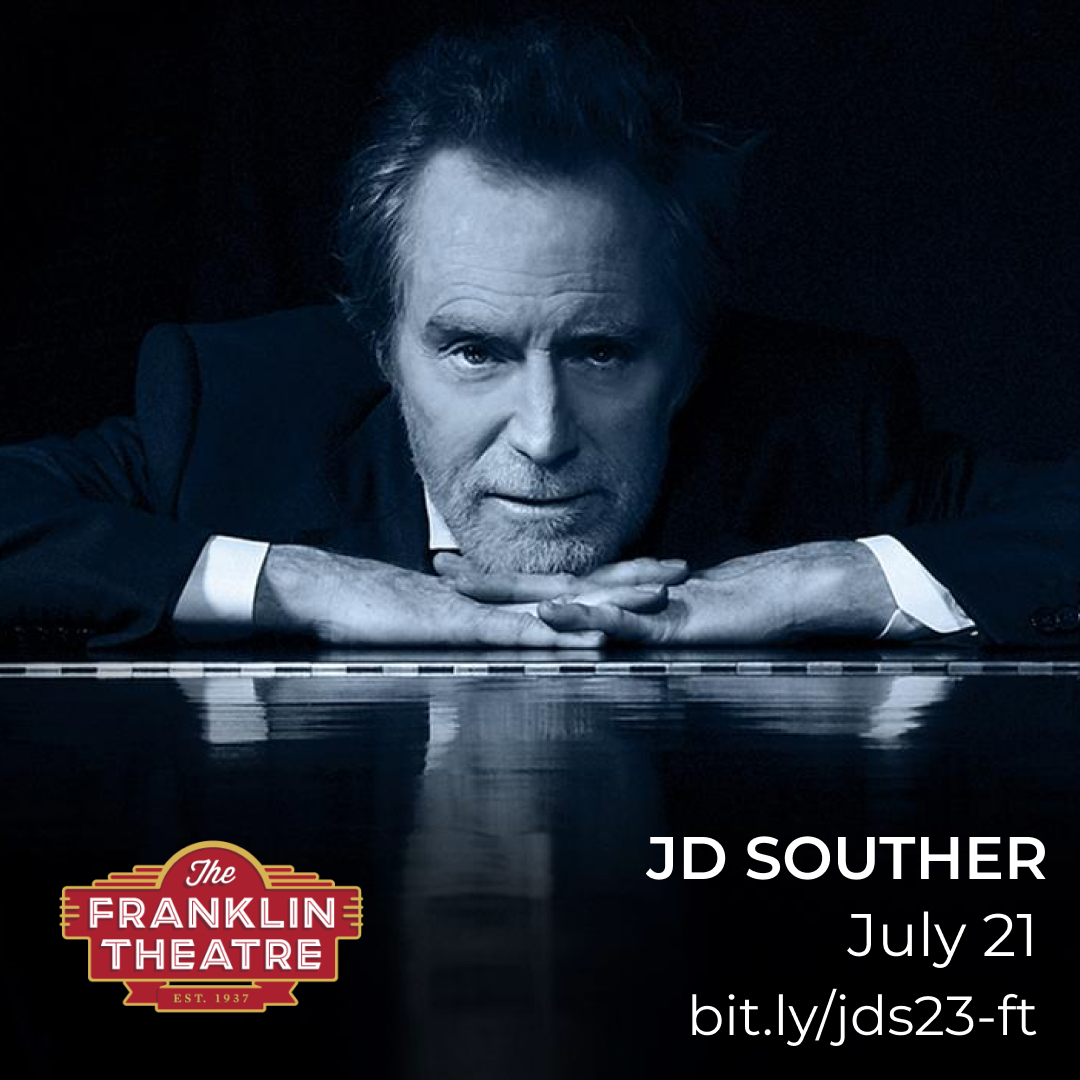This image is an advertisement billboard for the Franklin Theater, established in 1937. The top of the image prominently features J.D. Souther, an older gentleman with dark brown hair and slight stubble, implying he hasn't shaved in a few days. He is wearing a dark suit and is posed with his hands clasped together, resting on the top of what appears to be a piano, with his chin gently placed on his hands. His posture and expression have a direct, contemplative gaze towards the camera. The background is a rich, dark tone, adding a dramatic effect to the image. Reflecting on the glossy surface of the piano, his image is subtly mirrored. At the bottom right-hand corner, the Franklin Theater logo appears in bold, with the words "Franklin Theater" in large, white capital letters on a red background that resembles a theater marquee. On the opposite side, in white text, it states "J.D. Souther, July 21st," followed by a web link "bit.ly/JDS23-FT," providing details about the show.